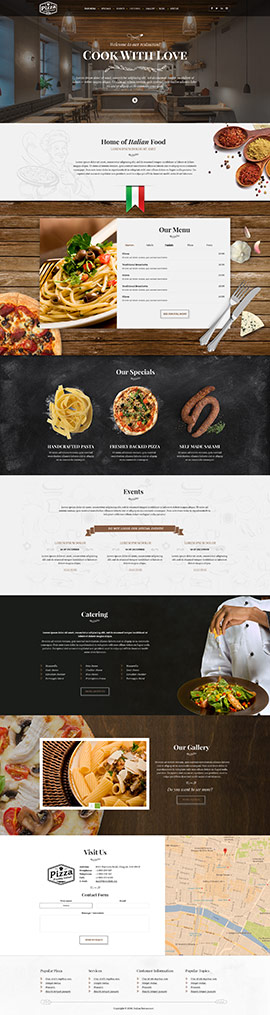A vibrant, detailed screenshot of a beautifully designed web page celebrating Italian cuisine. The webpage features a warmly lit kitchen backdrop with an evocative black banner displaying the phrase "Cook with Love" in elegant white lettering. The right-hand side is adorned with an array of aromatic spices, adding to the visual feast. At the center of the banner is the iconic Italian flag, its green, white, and red stripes proudly on display.

The menu, albeit small and slightly difficult to read, is garnished with exquisite silver cutlery—a fork and a butter knife—placed gracefully to the side. The food imagery is tantalizing: a wedge of white cheese accented with a touch of green, a plate of perfect pasta topped with fresh seasonings, and a mouth-watering pizza complete with savory toppings. Additionally, a portion of fettuccine is artistically spun at the bottom of the frame, accompanied by a delicious sausage.

Desserts also make an enticing appearance, and a substantial plate of large, rigatoni-like pasta commands attention at the bottom. For added cultural context, a map is incorporated, possibly highlighting regions of Italy known for their culinary specialties, completing this rich and inviting visual experience.